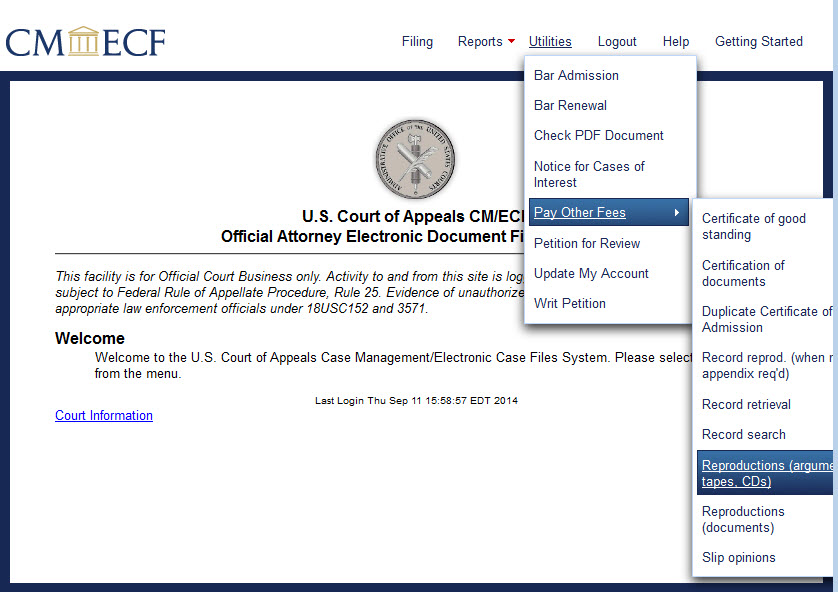The web page features a minimalist design with a white background and minimal color usage. At the top, in large, dark blue letters, the acronym "CME" is prominently displayed, followed by an icon representing a courthouse, and then the letters "ECF". 

Centered on the same top line are navigation tabs: Filing, Reports (with a dropdown menu), Utilities, Logout, Help, and Getting Started. The Utilities tab has been clicked, revealing a dropdown window with options including: Bar Admission, Bar Renewal, Check PDF Document, Notice for Case of Interest, and Pay Other Fees. The "Pay Other Fees" option is highlighted in a blue rectangle.

Clicking "Pay Other Fees" opens another window showing various services: Certificates of Good Standing, Certification Documents, Duplicate Certificate of Admission, Record Reproduction, Record Retrieval, Record Search, and an option highlighted under Record Reproduction as "Reproduction Documents".

In the center of the page, a letterhead states "U.S. Court of Appeals" and "CME ECF Official Attorney Electronic Document". A notice below indicates, "This facility is for official court business only."